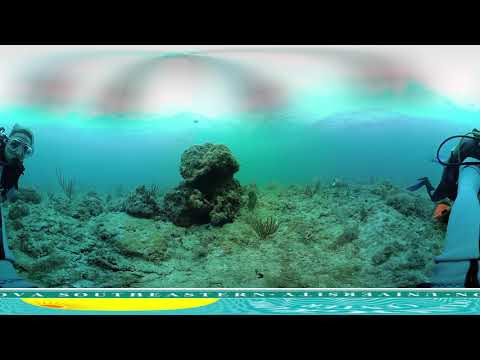The image features an underwater scene viewed through what likely appears to be a large window at a museum aquarium. Two scuba divers can be seen in the scene. On the left edge is a diver wearing goggles and a dark wetsuit, peering towards the center. On the right side, another diver is visible, equipped with full scuba gear including a tank, and appears to be holding a blue object. Central to the image is a large rock structure resembling a mushroom, extending from the bottom center towards the top. Surrounding the rock are various underwater plants and corals, with an overall color palette that includes shades of blue, green, tan, and black. The setting is rocky and algae-filled, suggesting a realistic underwater environment. At the bottom of the image, above a solid black border, a bluish-green banner with partially legible text includes words like "southeast" or "southeastern," though the full text remains unclear.